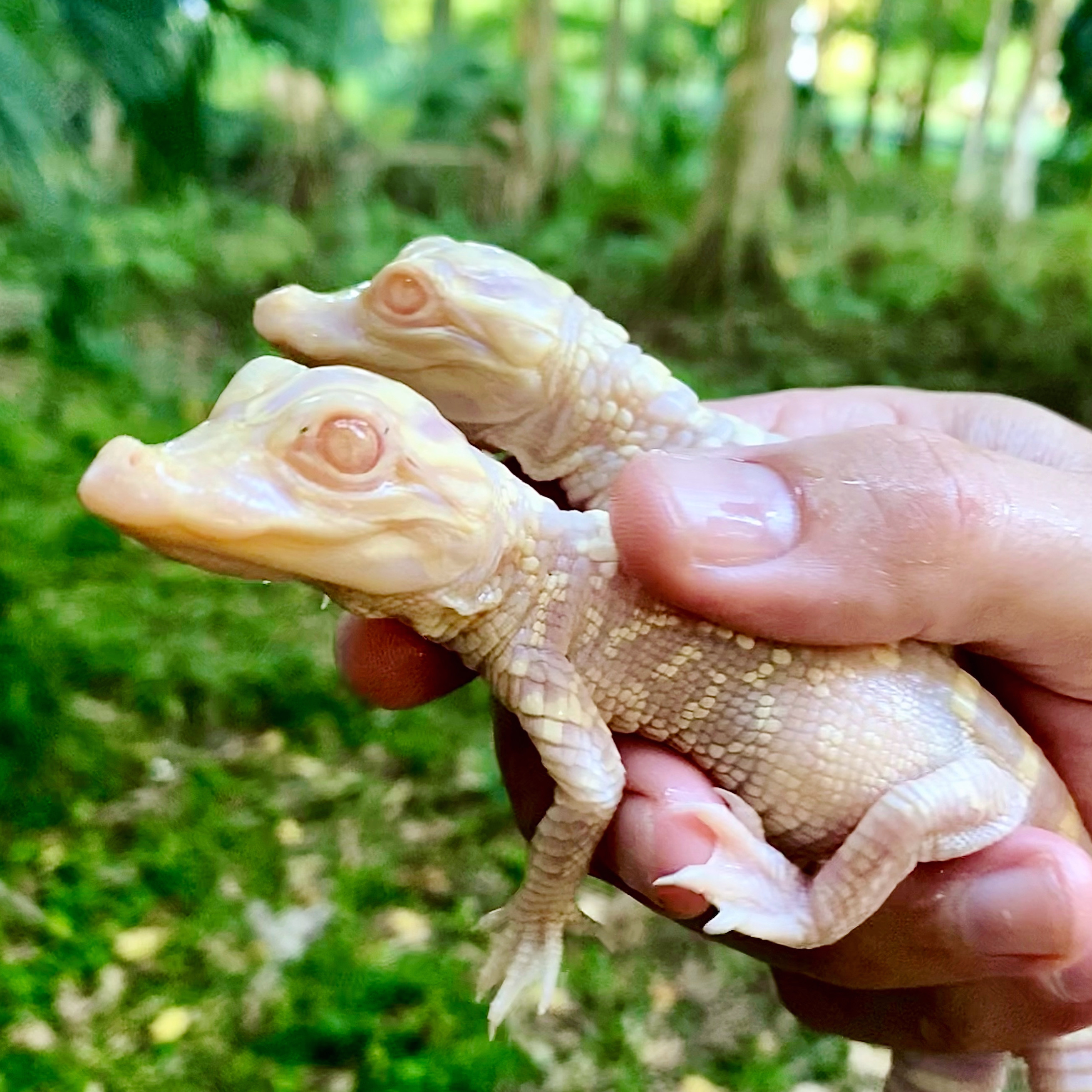The image is a detailed close-up photograph of a man holding two tiny baby albino alligators in his pale peach-colored hand. These small reptiles are characterized by their striking pale pink and white coloration, including their feet, claws, and scales. Their eyes are a delicate beige-yellow, a typical feature of albinos. One of the alligators is looking towards the right, while the other faces the camera, offering a clear profile view. The backdrop of the image reveals a lush, green forest, indicative of spring or summer, with rich green foliage suggesting that these rare creatures have just hatched in a season brimming with new life.